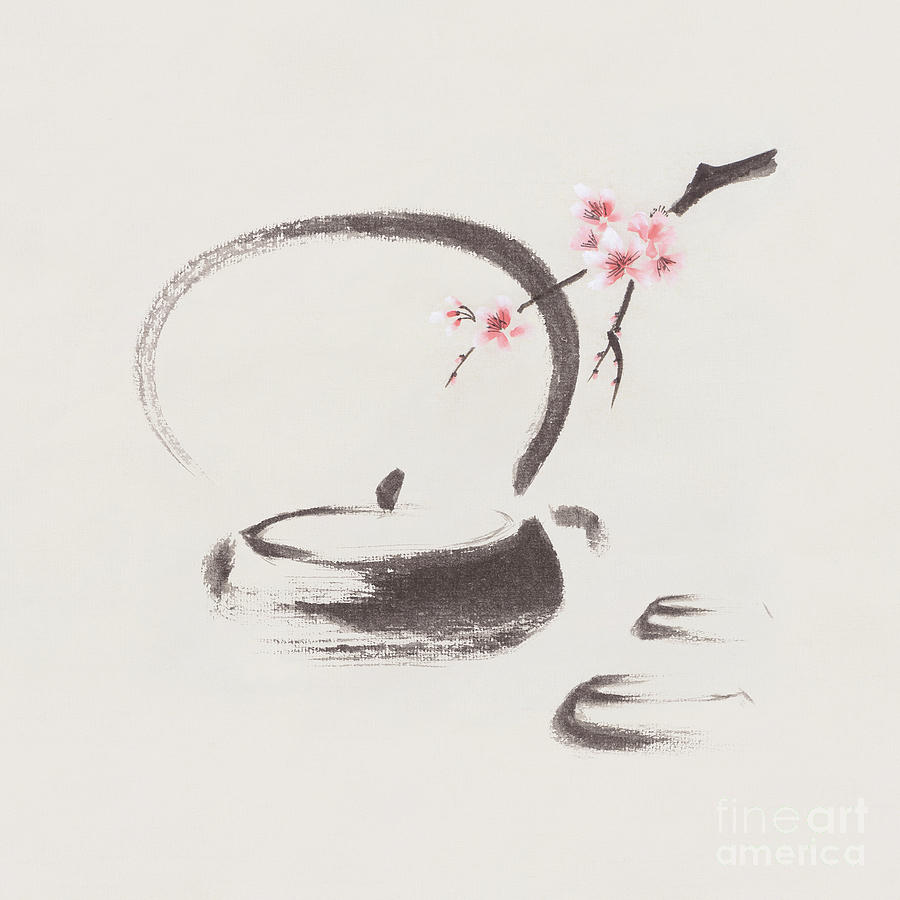This artwork, displaying Japanese influence, features a delicate and incomplete composition that blends elements of watercolor, ink, and charcoal. The scene unfolds on a subtle white canvas whose faint texture underlines the artistry's raw elegance. Dominating the top right corner, a sprig from a cherry blossom tree graces the canvas, adorned with pink and white blossoms in varying stages of bloom, infusing the piece with a touch of color and softness. Midway through the image, an indistinct teapot begins to emerge, its form loosely sketched with a grayish hue. The teapot includes a discernible handle and a subtle hint of a lid, suggesting its typical use for brewing tea. Accompanying the teapot, two small, unfinished cup-like shapes float nearby, adding to the ephemeral quality of the drawing. A dark smudge in the right corner and a black circle in the background add contrast and depth to the otherwise minimalistic scene. The watermark "Fine Art America" subtly identifies the piece as an item of refined artisanal origin, completing this intriguing blend of delicate lines and incomplete beauty.